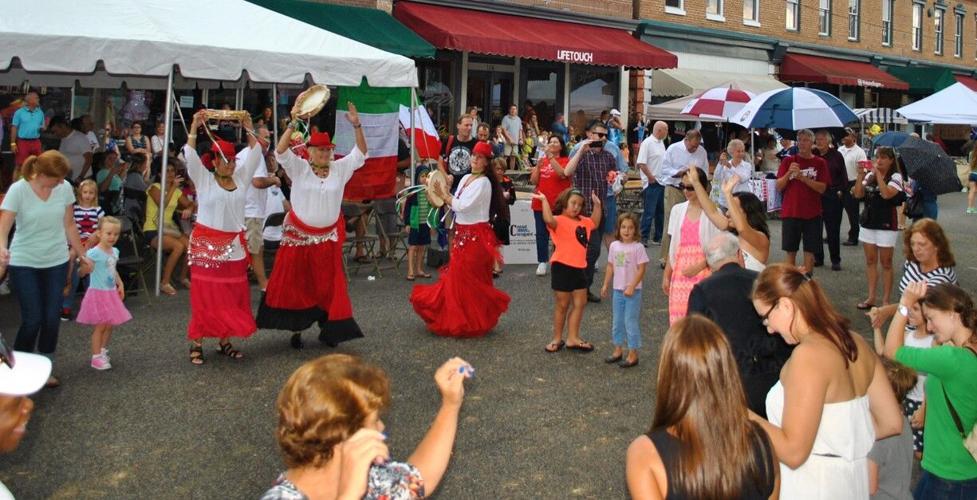In the image, a lively group of people is seen dancing in a circular formation in an outdoor setting during a festival. The event appears to be taking place on a gray-paved road. Central to the scene are three individuals dressed in red and white skirts, each playing a tambourine with one hand, except for the woman on the left who is using both hands to play her tambourine. The circle is composed of a diverse mix of women and children, all partaking in the joyous dance. In the background, a white tent is prominently displayed, adorned with a green, white, and red flag. To the right, a series of connected brown buildings are visible, featuring red and green overhangs. Additionally, a small white tent can be seen in the distance on the right side of the image, adding to the festive atmosphere.